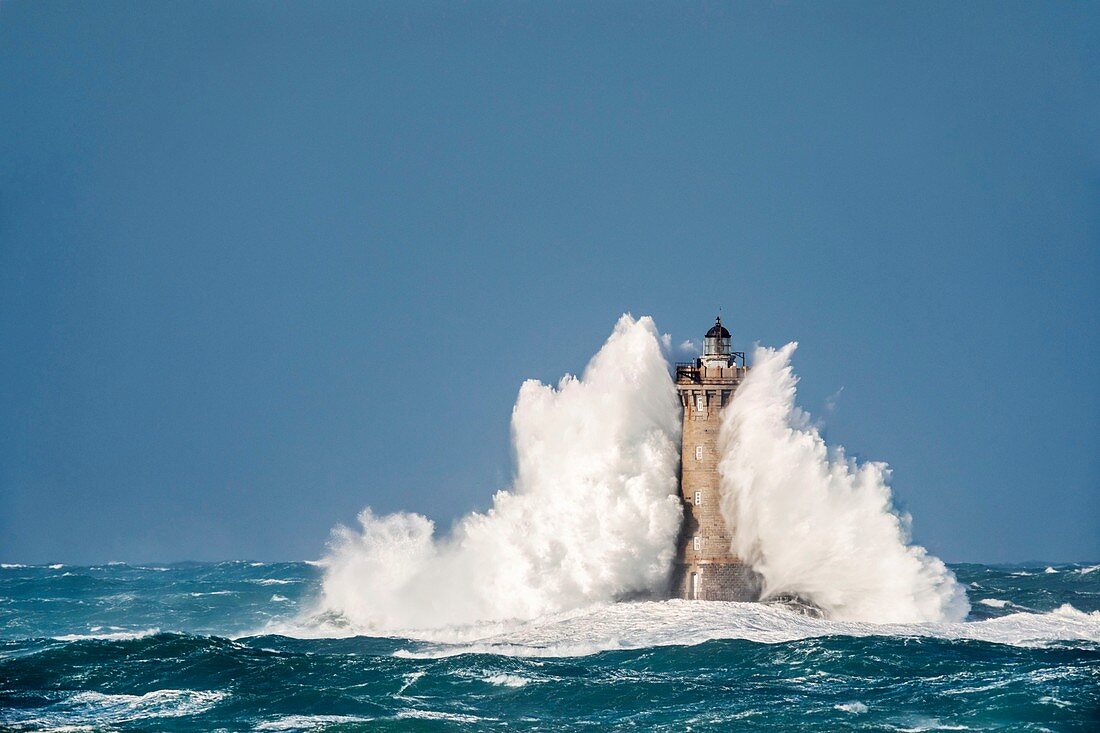The image depicts a solitary lighthouse set amid a vast, turbulent expanse of greenish-blue ocean, with waves surging and crashing violently around its base. The lighthouse stands resiliently on a concrete foundation partially visible beneath the pounding waves. Constructed from yellowish-beige and brown stone bricks, its structure tapers slightly as it rises. The exterior is punctuated by several tall, evenly spaced windows that ascend along its height. At the apex, a balcony equipped with a railing encircles the housing that contains the beacon light. The churning teal-colored ocean sends white-capped waves crashing up to the lighthouse's peak, almost engulfing it in a frothy embrace. This dramatic scene is framed by a perfectly blue, cloudless sky that stretches infinitely beyond the tempestuous waters, highlighting the lighthouse's isolation and resilience.